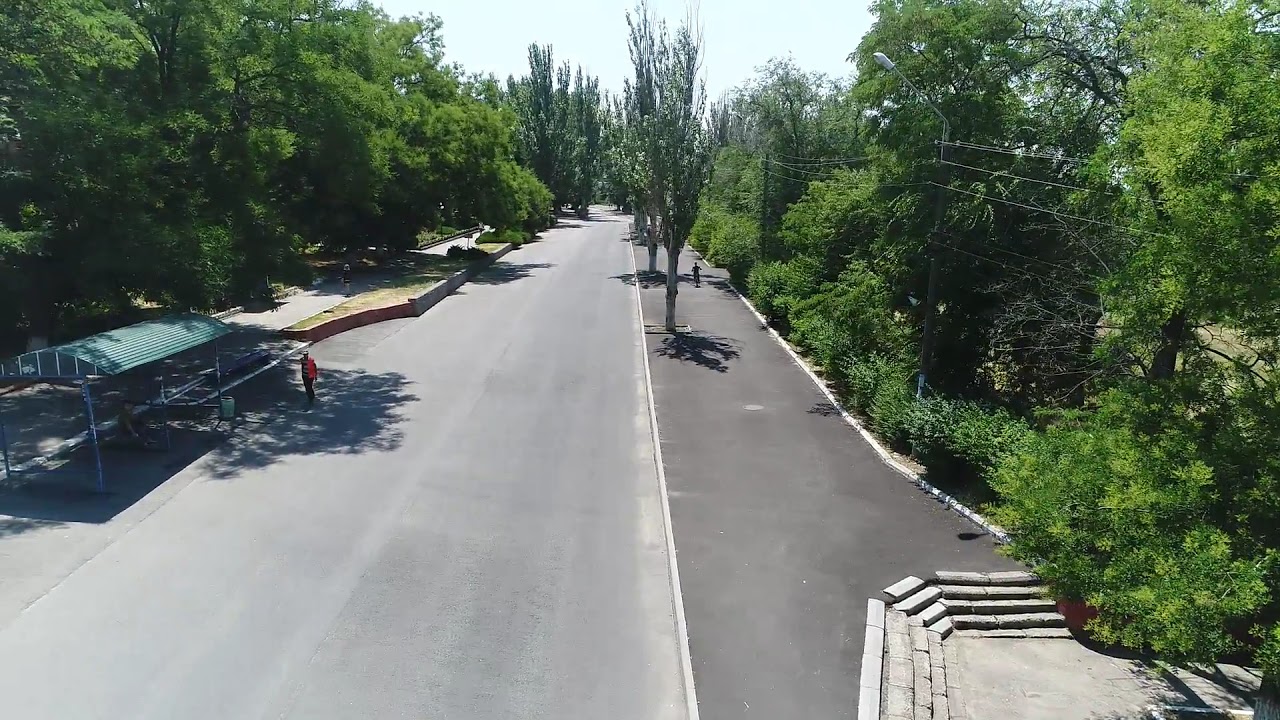The image captures a straight, long stretch of road, likely photographed from the second or third story of a building, possibly even by a drone given its angle. The road is flanked by dense, green trees with varying shapes and sizes. Along the road's left side, a temporary small green-covered awning or bus stop stands out, seemingly misplaced, potentially for an event like a marathon as it appears like a worker's station. A person in a striped shirt and red coat is walking towards this bus stop, where another individual is sitting on the ground. On the right side of the road, there's an unusually wide asphalt walkway, at least 10 feet across, sporadically interrupting the tree-lined area with small dirt patches for the trees. Electrical wires snake through the right side’s trees, and a set of steps descends into a partially visible path or park area. The road itself features a bump-out resembling a turn lane, and a typical sidewalk, also bordered by trees, runs parallel on the left. The coherent combination of natural and man-made elements, along with the scattered human presence, gives the scene a layered, almost preparatory ambiance.